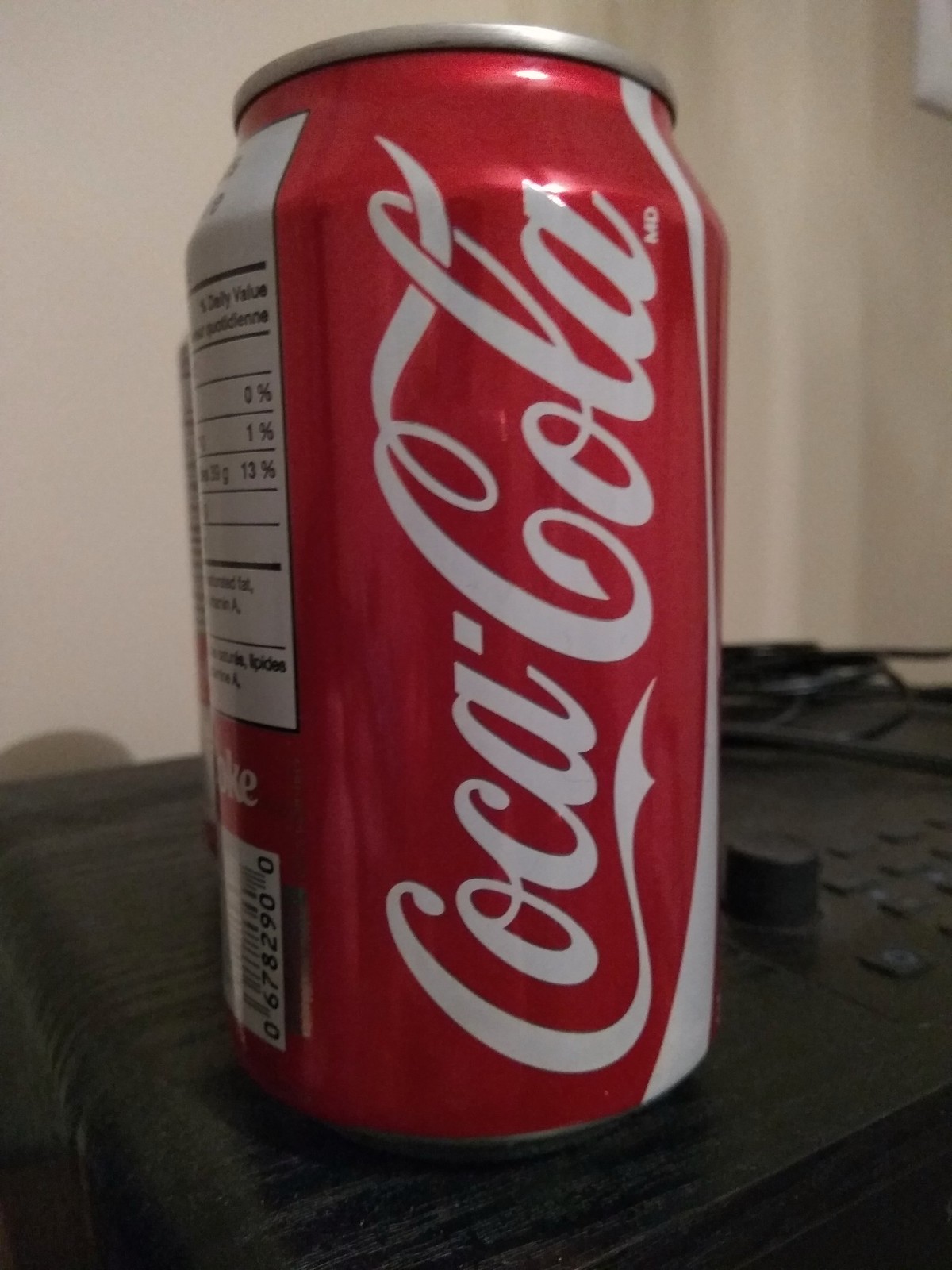This image features a very close-up shot of a classic 12-ounce Coca-Cola can, recognizable by its iconic red color and white cursive script logo, with a white stripe underneath the logo. The can is positioned vertically, and visible on the left side is a portion of the UPC code and nutritional information, although the details are somewhat obscured due to the angle. The Coca-Cola can is resting on what appears to be a wooden-textured surface with some electrical equipment, identified by the presence of knobs, buttons, and what seems to be a power button to the right of the can. Additionally, there is an electronic cord visible, suggesting the device is meant to be plugged into a wall. The background of the image is characterized by a plain white wall, making it difficult to ascertain the exact location or purpose of the setting.